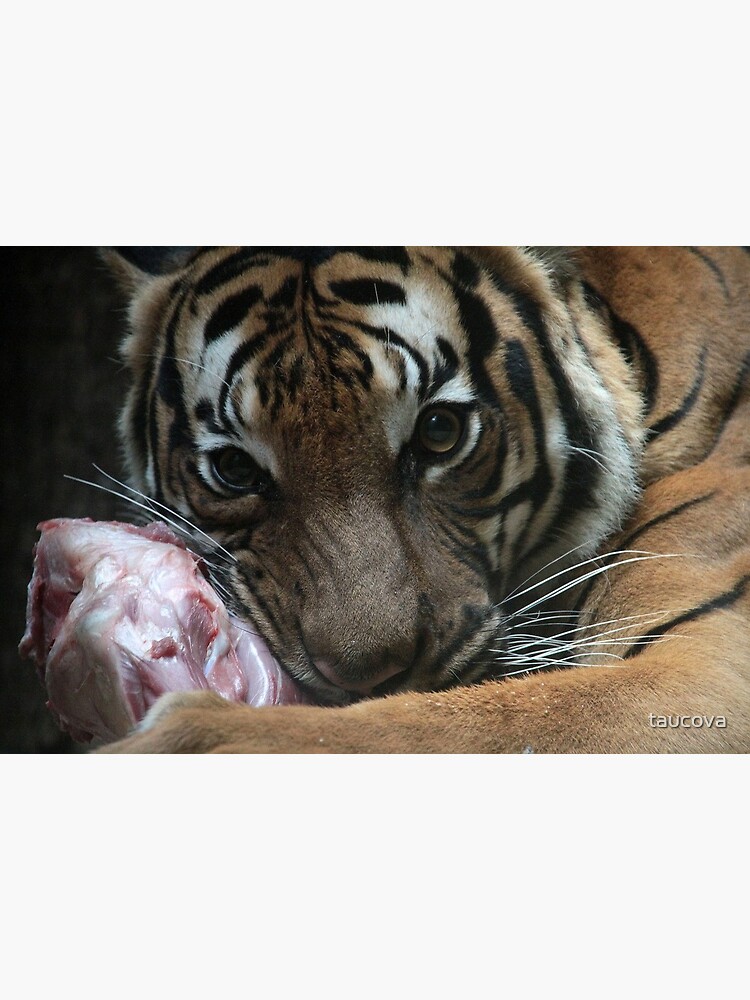This is a highly detailed, close-up photograph of a tiger's face, prominently featuring the textures and colors of its fur and the intensity of its gaze. The tiger's classic orange coat with striking black stripes and white accents around its eyes is captured vividly. Its large, expressive brown eyes are wide open with fully dilated pupils, suggesting a focused and intense moment. The tiger's nose is furrowed, and the right side of its mouth is scrunched as it bites down on a piece of raw meat, which appears pinkish with visible veins. This piece of meat, likely with a bone attached, is being held close to the tiger's face with its extended left paw, indicating that the tiger is laying down. The large white whiskers of the tiger rest against the meat, adding to the intricate details of the photograph. At the bottom right-hand corner of the image, the word "Tacoba" is visible, providing a textual element to the scene. The overall composition emphasizes the tiger's natural beauty and the primal act of feeding.